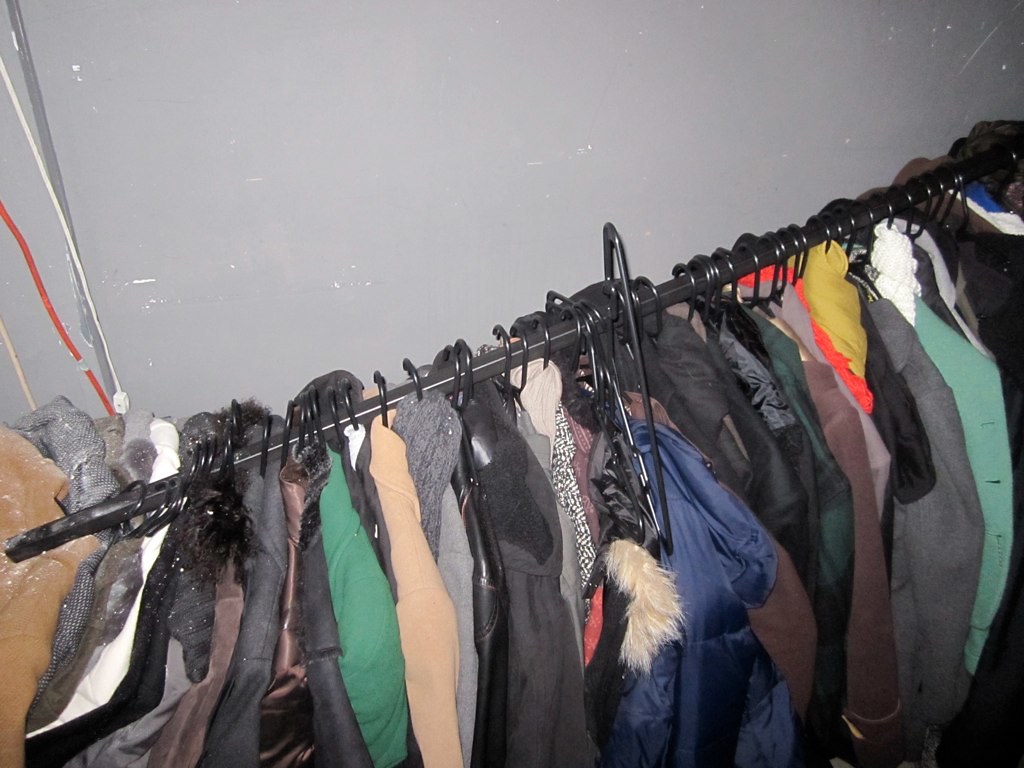This is a detailed aerial colour photograph taken from inside a closet. The image captures a black clothing rack, running almost diagonally from the lower left to the upper left corner, filled with over 30 assorted garments hanging on black hangers. Behind the clothes, the wall appears grey and scuffed with white flecks or scratches. On the left-hand corner, there are visible cords in red, yellow, white, and possibly a brown area that might be cardboard.

The clothes are predominantly coats, exhibiting a wide range of colours including black, brown, green, beige, grey, blue, red, yellow, white, and teal. Some specific details include a garment with a black and white print, a blue coat with a furry hood, and a green jacket with visible buttonholes towards the left. The overall scene hints at an untidy environment, with white plaster dust scattered on the tops of the coats and even on the black bar. One of the hangers is askew, suggesting a possible disturbance or fall of the rack.